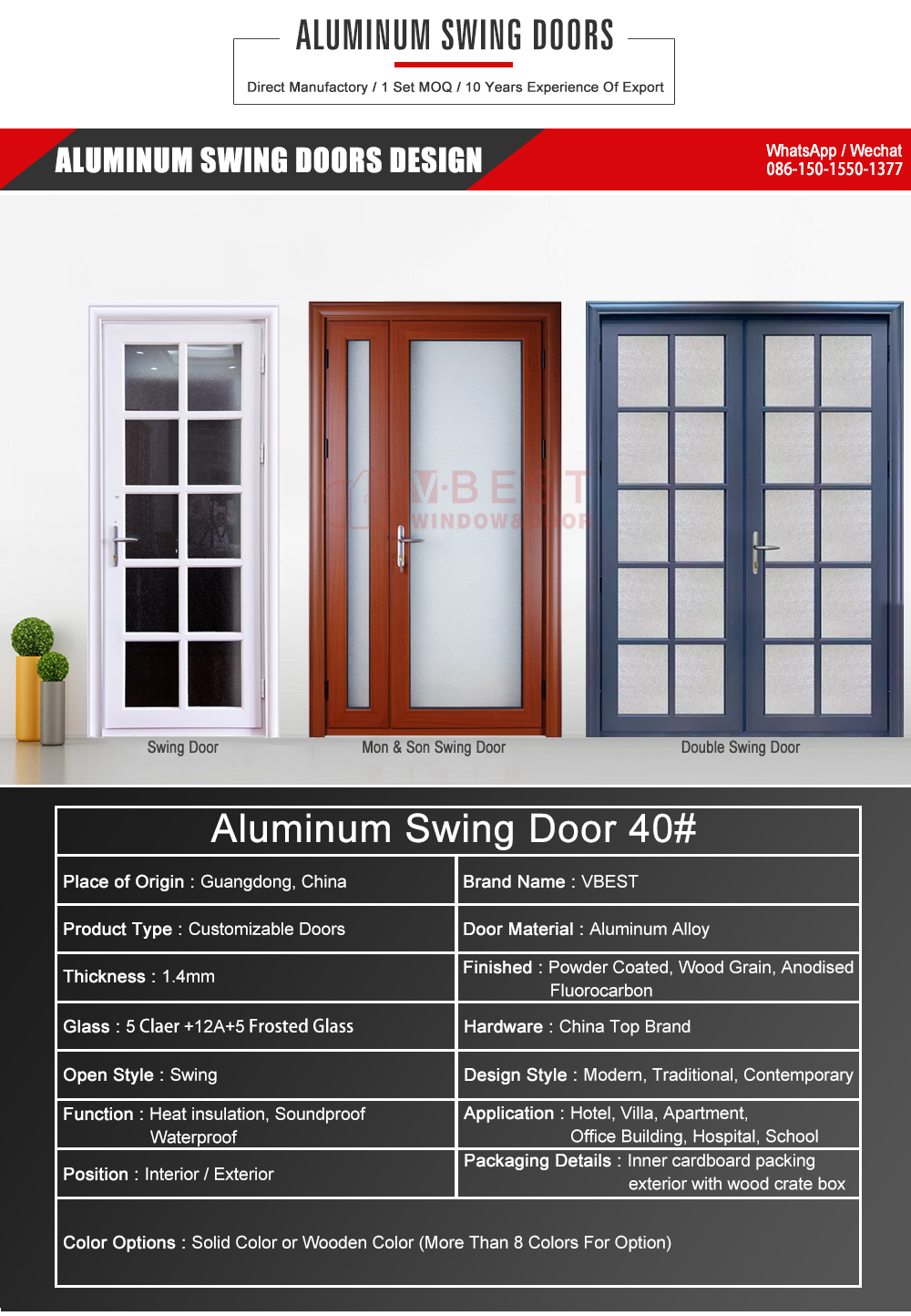The brochure showcases aluminum swing doors offered by the company, emphasizing their various features and customization options. The rectangular brochure, measuring approximately 5 to 6 inches high and 4 inches wide, features a prominent header at the top with bold black print stating "Aluminum Swing Doors" on a white background. Positioned to the left and right, there are red and black bands, with the right-hand side containing contact information for WhatsApp and WeChat.

Beneath this, a thin black pinstripe creates a rectangle framing more detailed information about the company, which boasts "Direct Manufacturing," a minimum order quantity (MOQ) of one set, and "10 Years Experience of Export." Below this header, a white background showcases three types of aluminum swing doors: 

1. The door on the left is white with ten small, square, gray panes of glass and labeled as a "Swing Door."
2. The center door, a "Mon & Son Swing Door," features frosted white glass framed by cherry wood.
3. On the right is a blue double swing door with ten panes of frosted glass on each side.

The lower section of the brochure details the technical specifications, including the product type (Customizable Doors), place of origin (Guangdong, China), door materials (aluminum alloy), thickness, open style, function, position, color options, brand name (V-Best), hardware details, design styles, applications, and packaging details. The comprehensive layout ensures potential customers have all the necessary information to make an informed decision about their purchase.